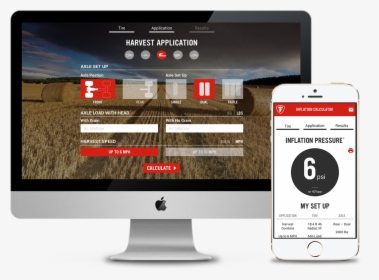The image displayed on a computer screen features a picturesque scene of a field with bales of hay, characterized by a rich brown landscape at the bottom and a vibrant blue sky adorned with a scattering of clouds at the top. Superimposed on this background, the words "Harvest Application" are prominently shown in white. Additional information related to the application and its functionalities is also present but not legible due to its small size. To the side, the interface depicts a silver smartphone showcasing key data points relevant to the harvest application, including fields labeled "Application Time," "Application Remarks," and "Inflation Pressure." The inflation pressure is highlighted within a black circle in white numbers, displaying "6 PSI." Below this section, the phrase "My Setup" is also visible in black text. The Apple all-in-one computer sits on a pristine white table. The screen's contents detail various tire conditions and specifications, crucial for agricultural purposes, as evidenced by the visual and numerical indicators such as the 6 PSI reading related to tire pressure.